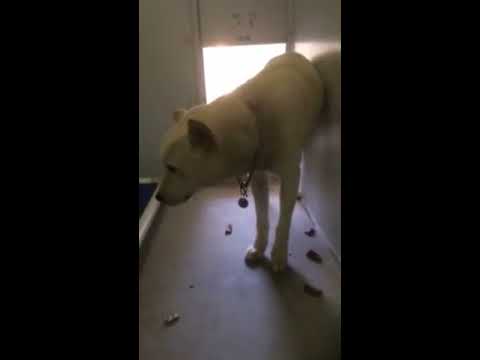In the center of the image, we see a short-haired white dog with black ears, wearing a collar that features a circular medallion. The dog is positioned such that its front legs are visible, while its back legs and tail are obscured, seemingly still partially inside a dog entrance. The dog is looking to its left, which is our left. Surrounding the dog, there are scattered items on the floor that could either be treats or small piles of poop, adding a sense of disarray to the scene. The background suggests this might be a kennel or animal shelter, indicated by the white walls and a small, illuminated square opening. The floor is a similar whitish color to the walls, and there's a blue area beside the dog. The left and right thirds of the image are bordered by black bars, giving the scene a framed appearance. A small black container is also visible on the left edge of the image.